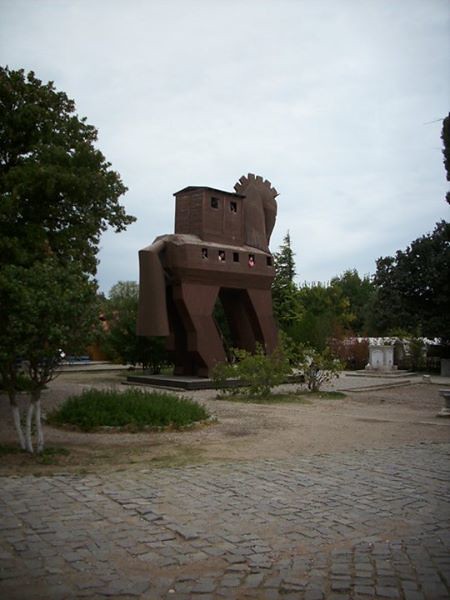The photograph captures a large, sculptural monument that draws the viewer's attention immediately. The structure, reminiscent of a large horse, appears to be constructed from metal and includes multiple windows, from which small figures or people seem to be peeking out. The horse-like monument features details such as stylized legs, a head, and a tail, and there's a tower or barracks-like element integrated into its design. The dark brown to blackish structure stands within a manicured park setting, surrounded by cobblestones and brick tiles, with patches of short green shrubbery and grass. Trees with bushy green leaves frame the scene on the left and in the background, while the sky above is overcast, filled with white clouds that obscure the sun, creating a subdued daylight atmosphere.